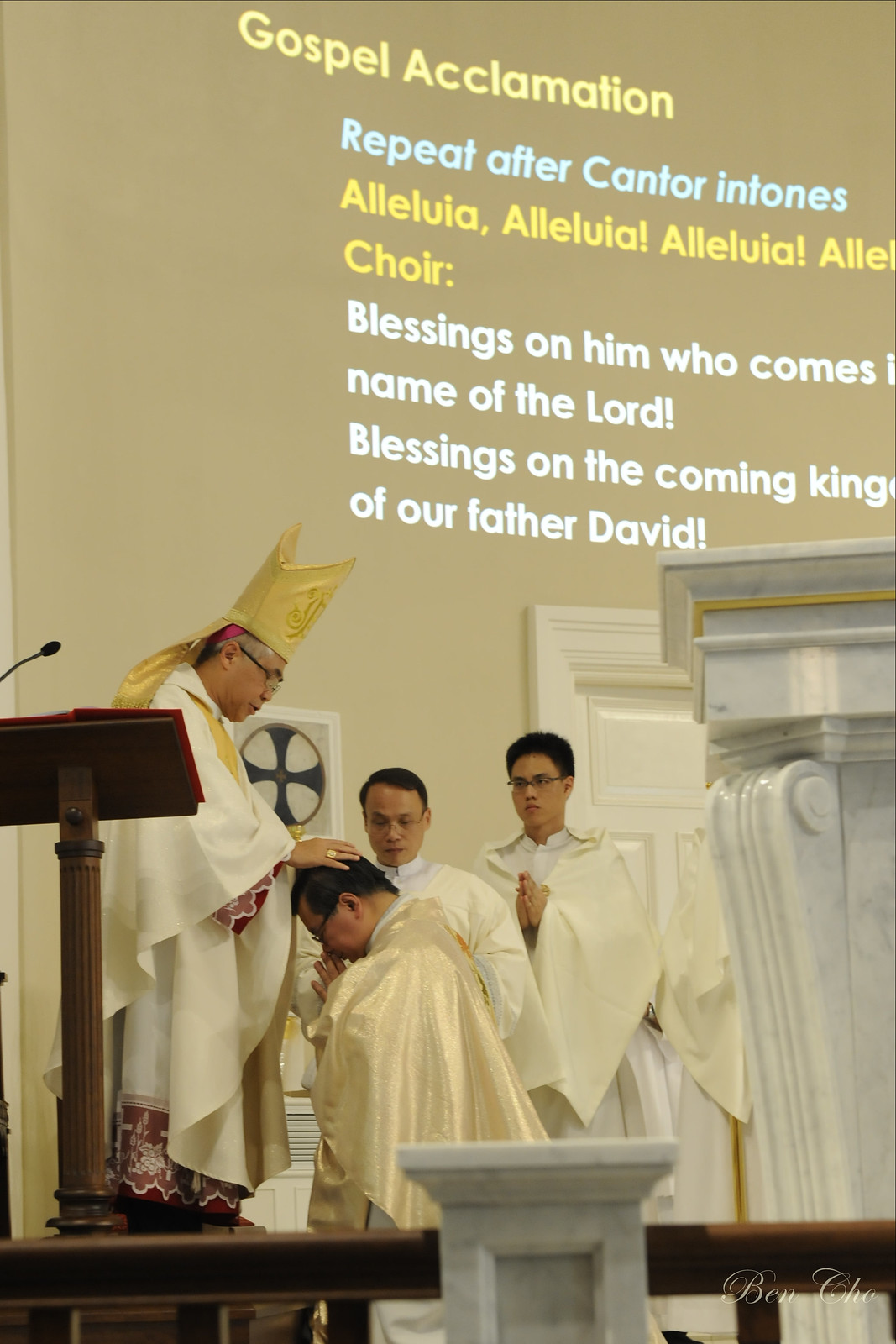The image depicts a solemn scene inside a church, featuring a rich blend of religious and cultural elements. At the top of the image, bright yellow text proclaims "Gospel Acclamation," followed by the instructional "Repeat after the cantor in tones" printed in blue. Below, the word "Alleluia" appears four times, also in yellow. Interspersed within is white text delivering blessings: "Blessings on Him Who Comes, Name of the Lord, Blessings on the Coming Kingdom of our Father David."

A man, who appears to be a high-ranking clergy member, possibly the Pope, is featured prominently on the left side of the image. He is adorned in an ornate white robe and a golden hat, placing his hand on the head of an Asian man kneeling in prayer. This scene suggests a moment of blessing or anointment.

Adjacent to this central interaction, a line of Asian men, dressed in robes and hands in prayer, look down reverently. They are situated in front of a brown wooden podium that holds a book and a microphone. The surrounding room has a beige, high-ceilinged interior, highlighted by a white door and a gray column with a gold stripe across its top. Marble elements add to the ecclesiastical setting. The text and the solemn activities collectively pronounce a moment of religious significance within the church.